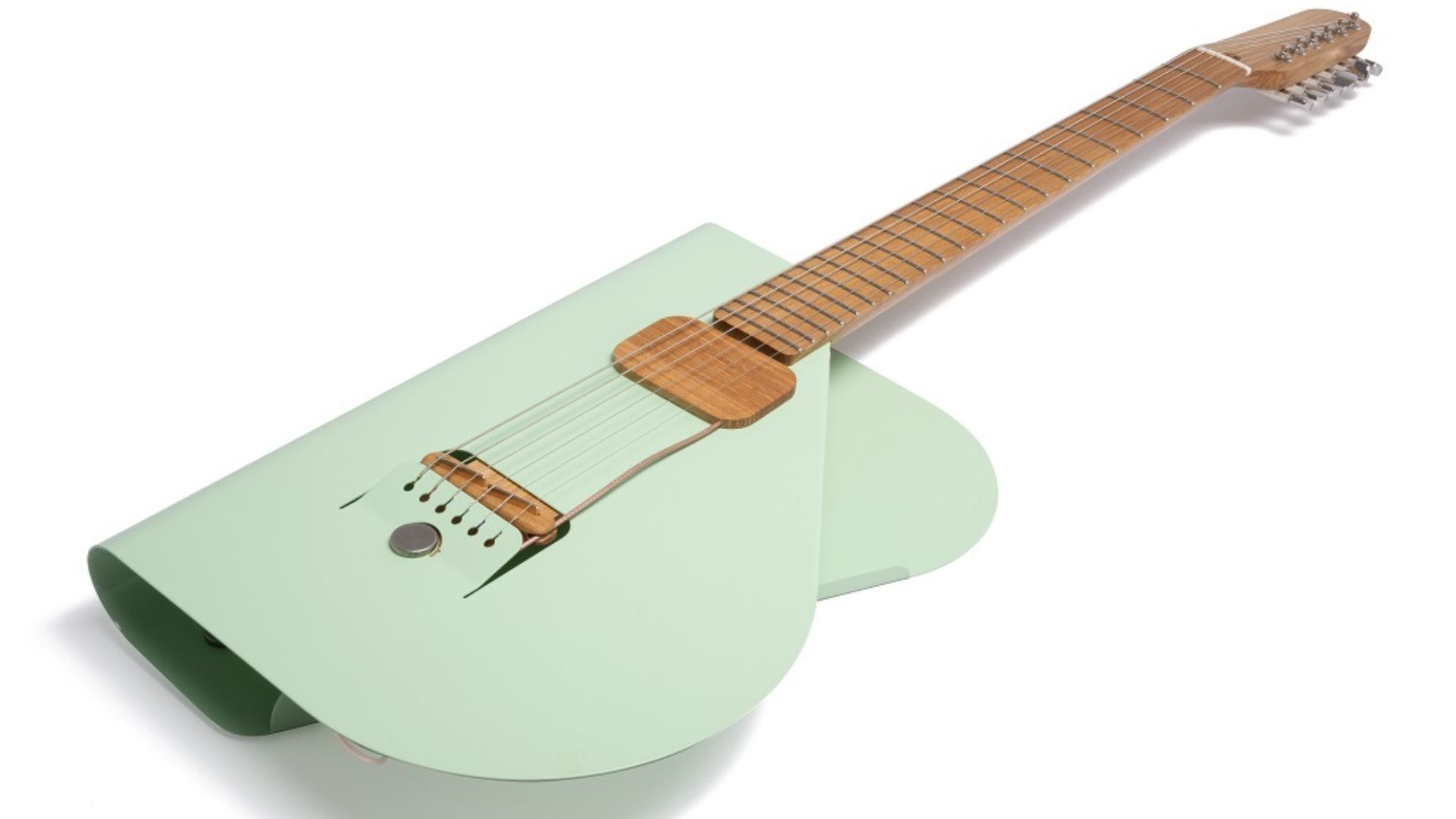The image features a unique guitar seemingly handcrafted from construction paper or a sturdier type of paper. The guitar has a distinctive design with a wooden-like fretboard and a thin, mint green body that appears folded in half, creating a smooth, seamless edge without any visible crease. The colors on the guitar include mint green, white, gray, and a wood-like mahogany hue. The guitar is positioned diagonally, with the base pointing towards the bottom left corner and the neck extending towards the top right. The background is a stark, empty whiteness, highlighting the guitar as the central focus. This artistic creation lacks any text or writing, adding to its minimalist and clean aesthetic.